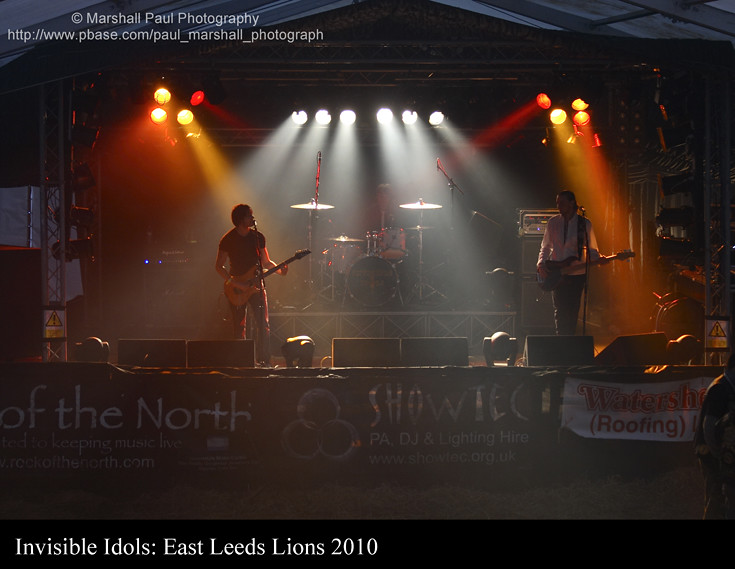The image captures a live concert featuring the band Invisible Idols during the East Leeds Lions 2010 event. The stage is outdoors, partially covered by a white tarp, and brightly illuminated by multi-colored lights, including prominent orange and red hues. At the forefront, the banner "Invisible Idols, East Leeds Lions 2010" is visible in white text. Additionally, there are various promotional signs: "Waters Roofing," "Showtech Lighting," and "rockofthenorth.com" which states "Keeping Music Live."

On the stage, the left guitarist, donning a black t-shirt and jeans, passionately sings while playing a yellow guitar. On the right, the bass player sports a white long-sleeved shirt and wields a black bass. Centrally positioned, elevated on a riser, the drummer is partially visible behind a white drum set with dual cymbals on each side and a black bass drum. Notably, tall speakers flank the stage edges, enhancing the live music experience. The upper left corner features a credit for the photographer: "Marshall Paul Photography," with a web address. The performance atmosphere is energetic, captured under the vibrant light show, contributing to the overall dynamic evening scene.